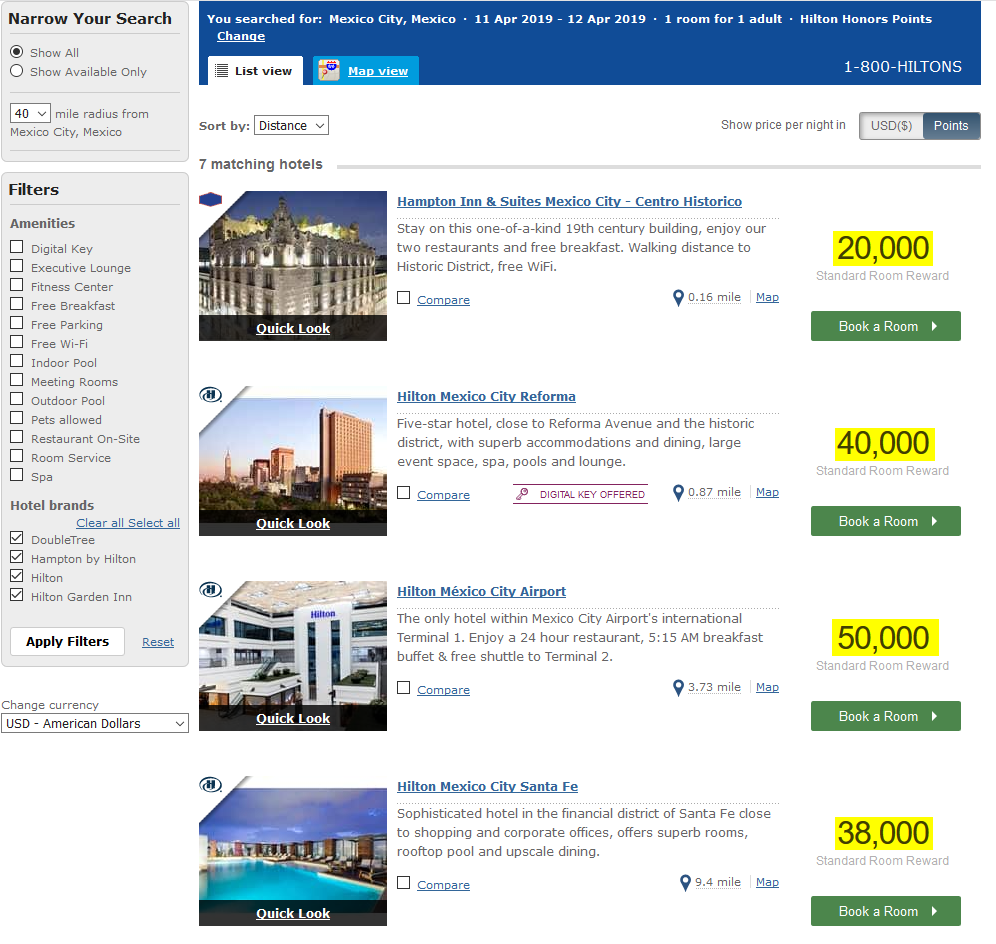On a travel website designed for booking hotels, a detailed filtering system is available on the left-hand side to help you narrow your search. The filters allow you to refine your search by criteria such as availability ("Show all" or "Show available only") within a specified radius, starting from a default of 40 miles from Mexico City. This radius can be adjusted via a pull-down menu. 

Further, you can apply filters based on various amenities including a digital key, executive lounge, fitness center, free breakfast, free parking, free Wi-Fi, indoor pool, meeting rooms, outdoor pool, pets allowed, restaurant on-site, room service, and spa. Though none of these amenities are pre-selected, users can choose based on their preferences. 

Under the hotel brands section, checkboxes show selections for Doubletree, Hampton by Hilton, Hilton, and Hilton Garden Inn, all of which are checked. There are options to clear all selections, apply filters, or reset everything. Additionally, the site allows for currency exchange, with USD as the default currency.

At the top right of the website, it indicates that you searched for hotels in Mexico City for a stay from April 11, 2019, to April 12, 2019, requiring one room for one adult using Hilton Honors Points. There’s an option to change these search criteria. The interface includes two viewing tabs: "List View" (which is currently selected) and "Map View."

The search results are sorted by distance and display prices in USD. Seven hotels match the search criteria. The top-listed hotel is Hampton Inn and Suites, Mexico City, Central Historic District, which costs 20,000 points for a standard room.